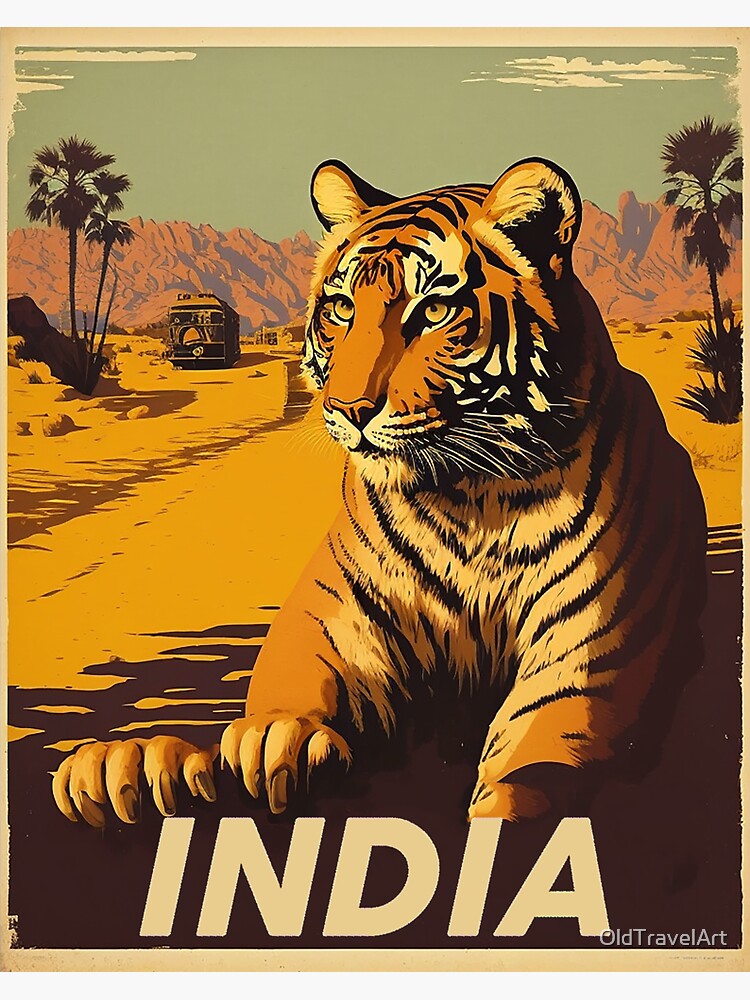The vertical cartoonette poster features a vividly drawn, majestic tiger in the foreground, slightly right of center. The tiger—adorned in striking orange and black stripes, with expressive eyes and touches of yellow—is lying down with its right paw prominently displayed and its left paw disappearing behind the large, white letters spelling "India" at the bottom. The artwork is framed by a light tan border. The backdrop depicts an arid landscape with rocky terrains, scattered palm trees, and a traditional Indian vehicle visible on a distant path leading to orangish-brown mountain formations. Above this scenic desert ground, the sky transitions into a blue-gray hue with soft, white clouds. Subtly blending warm tones for the natural environment and cooler tones for the sky, the poster captures an evocation of the Indian landscape under a clear sky. In the bottom right corner, the inscription "old travel art" stands out, adding to the overall vintage aesthetic of the poster.